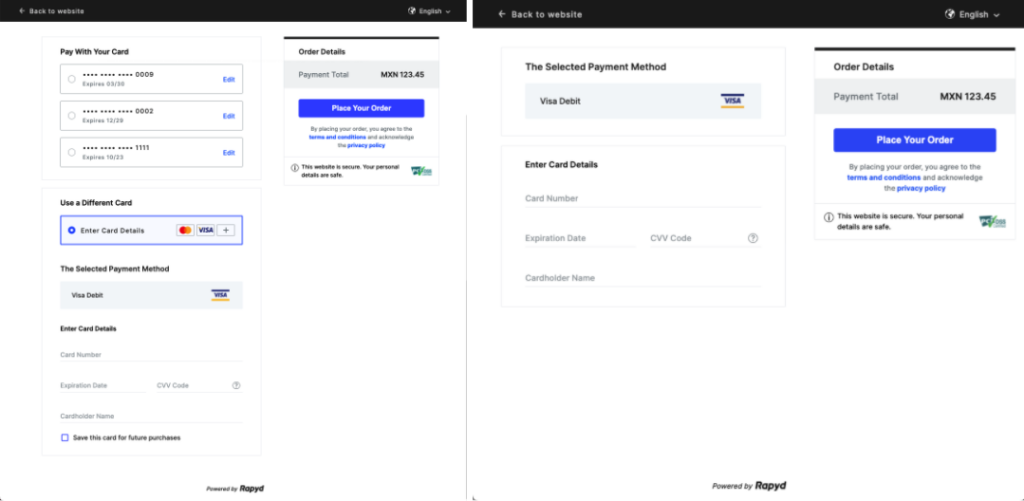This image features a comparison of two screenshots from the final stage of a website payment process. On the left side, the user is prompted to select a payment method, displaying three available cards, including a Visa Debit. Below these options is an alternative to "Use a different card" which, when selected, allows for manual entry of new card details. The right-side screenshot mirrors this setup, showing the same Visa Debit card as the selected method. Notably, the card details in both screenshots remain unentered. The order summary at the bottom confirms a payment total of MXN 123.45, which appears to be a sample amount rather than a genuine transaction.